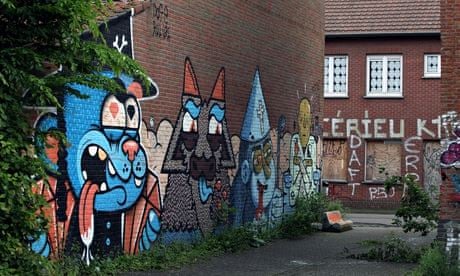This photograph captures an alleyway in a residential area adorned with vibrant graffiti. Dominating the scene is the side of a tall, somewhat dusty brown brick building on the left, where most of the artistic action is concentrated. The brick wall is interspersed with patches of foliage at the far left edges and the bottom, adding a touch of nature to the urban setting.

The graffiti features a series of colorful, blue-skinned characters seemingly straight out of an animated world. On the left, there's a quirky figure with the combined appearance of a dog in a European-style cop uniform, marked by his distinctive eyes—one pink, one black—both diamond-shaped, and his tongue sticking out with drool. Next to him is a fantastical creature that merges elements of a wolf and an owl, sporting triangular features, red pointy ears, blue eyebrows, and a black-and-blue tongue.

Further along, we encounter a blue monkey with striking white facial hair, wearing a light blue party hat. The monkey’s quirky personality is showcased through a pipe in its mouth. The final character is a man depicted in a straight jacket or perhaps a lab coat, adding an element of mystery to the ensemble. Behind this character, the adjacent building features graffiti reading "DAFT" along with other indecipherable texts like "C E R I E U" and "E R P," all splashed across its boarded-up windows.

The alley itself consists of a gray asphalt road with grassy borders, framing the visually captivating art display. The contrast between the artistic mural and the rundown environment highlights both the creative and gritty aspects of urban life.